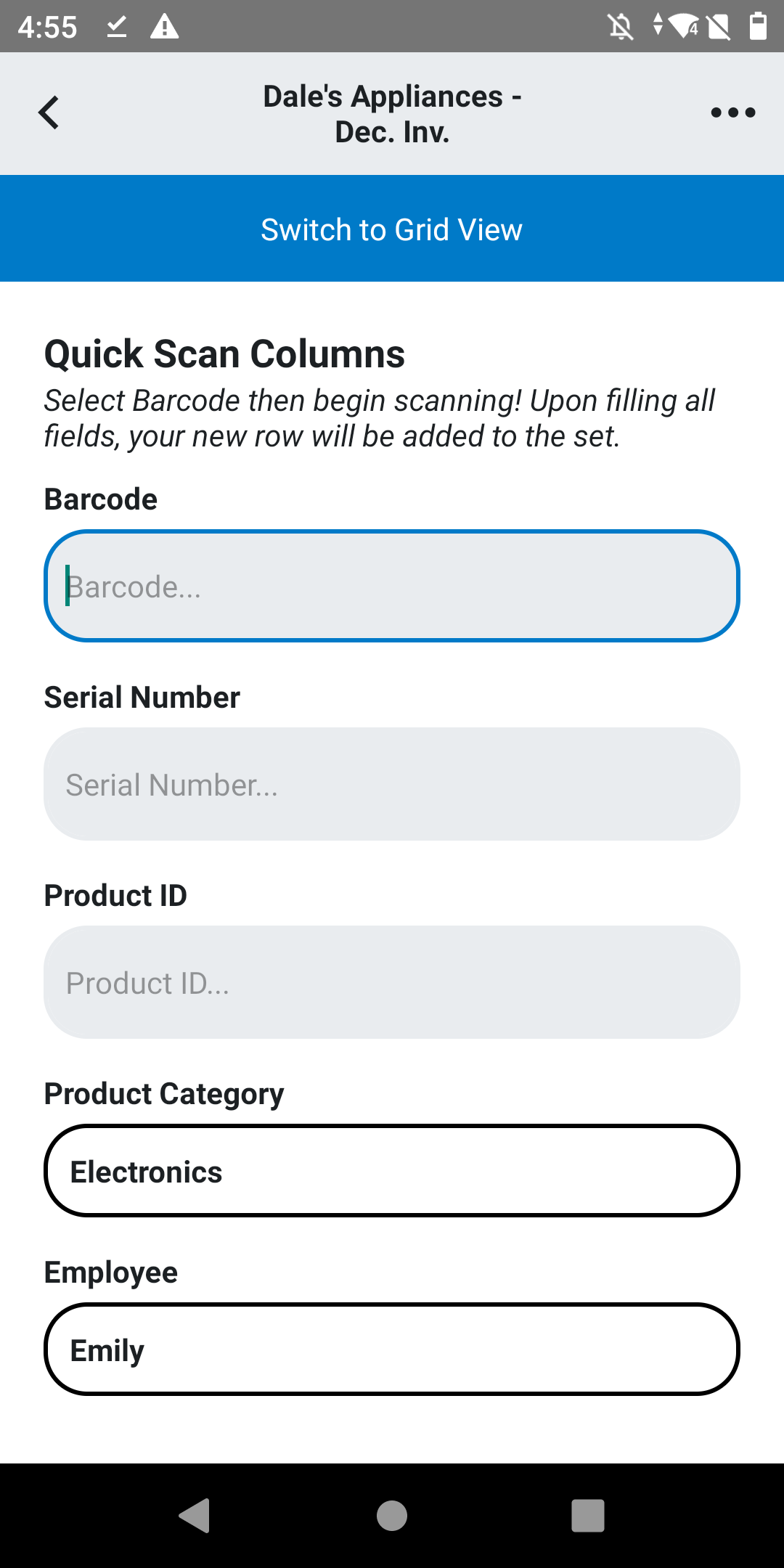This image depicts a minimalistic app interface for Dale's Appliances, possibly for conducting a December inventory (DEC.INV). At the top of the phone screen, the status bar displays the time as 4:55, accompanied by a check mark, an alert notification triangle, and an indication that the alarm is turned off. Wi-Fi signal strength and battery level are also visible.

The main interface header reads "Dale's Appliances, DEC.INV" and features a blue bar prompting users to "Switch to Grid View." Below this header, there are options for "Quick Scan," "Column," "Select Barcode," and "Begin Scanning." Instructions are provided, stating that upon filling out the fields, a new rule will be added to the set.

The barcode entry section includes a large, empty input field outlined in blue, with a cursor marker indicating readiness for typing. Below the barcode field, there are additional empty fields labeled "Serial Number" and "Product ID," both with gray backgrounds indicating that no text has been entered yet.

Further down, the app shows "Product Categories: Electronics" and lists "Employee: Emily," suggesting that Emily is responsible for scanning barcodes in the electronics category for the December inventory. The interface concludes with a navigation menu at the bottom of the screen.